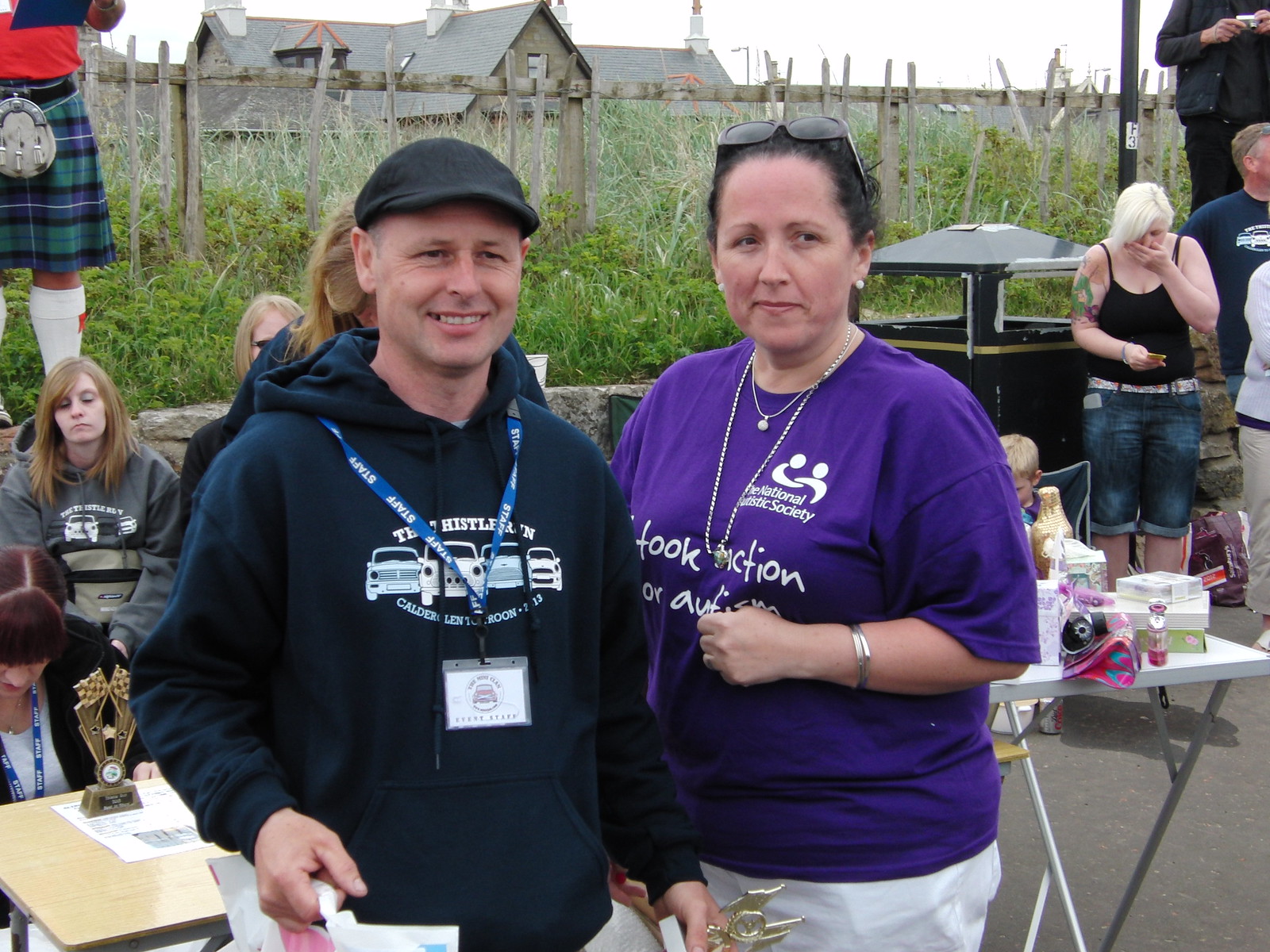In this large square photograph taken outdoors on an overcast day, a diverse group of people is captured at an event. At the forefront, a smiling man stands on the left, wearing a black hoodie adorned with car designs, a black cap, and a blue lanyard. He holds a bag in his right hand and what could be the top of a trophy in his left. Next to him is a slightly heavyset woman with dark hair pulled back, glasses atop her head, wearing a purple shirt with white lettering supporting autism, and light-colored pants. She accessorizes with a long necklace chain, a shorter necklace with a small pendant, and a bracelet on her left arm. 

In the background, the scene is populated with people and various items on tables, against a backdrop of green shrubbery, a short stone wall, and a wooden fence. Notably, a woman with short bleach blonde hair, wearing denim Bermuda shorts, a sleeveless tank, and sporting a large tattoo on her right arm, has her left hand over her mouth. Nearby, a small child sits in a chair. On the left side, visible is a trophy on a table, a woman with a lanyard looking down, another woman with a board expression sitting behind her, and the bottom half of a man standing on the stone wall in the upper left corner. This man is clad in tall white socks and a plaid kilt of blue, green, and black. The overall ambiance suggests a communal gathering, possibly a fundraiser or awareness event, with bright light filtering from the white sky above.